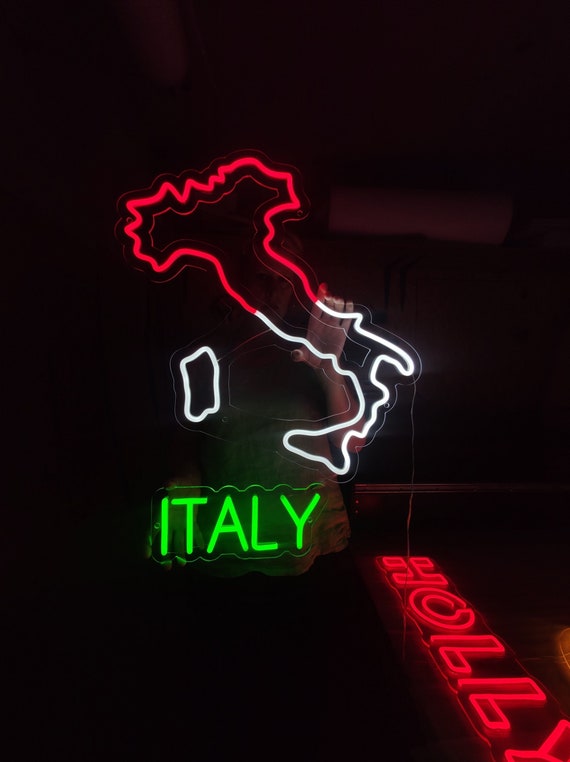In a dimly lit indoor setting, the color photograph captures a person standing in the darkness, barely visible save for the faint outline of their short-sleeved light blue shirt. They are holding up a neon sign with their left hand. The sign depicts the boot-shaped outline of Italy, its top section illuminated in red while the lower part glows white. Accompanying this outline, the word "ITALY" appears in vibrant green neon lettering at the bottom. To the left of the boot, the island of Sardinia is outlined in white. On a table to the right side of the image is another neon sign that flashes the name "HOLLY" in red, positioned vertically. Although the person's features are obscured by the darkness, the illuminated neon signs cast a captivating glow that highlights the striking contrast between the colors and the surrounding shadows.